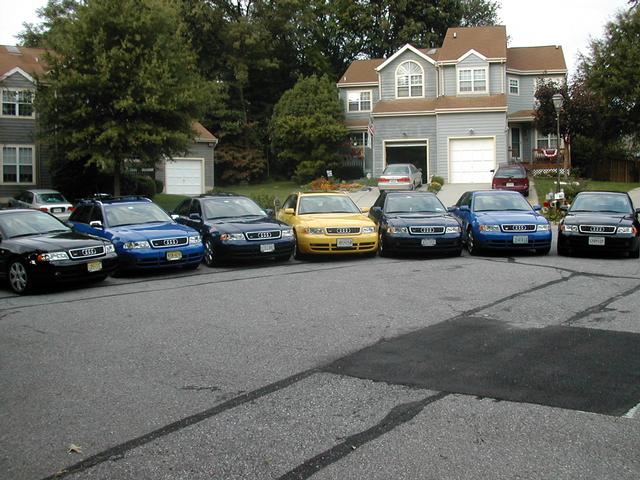In the photograph, a collection of seven late-model Audi four-door sedans is meticulously lined up in a cul-de-sac, which forms part of a quiet neighborhood. The cars are arranged in a distinctive pattern, alternating between black, blue, black, yellow, black, blue, and black. This display is set against the backdrop of two grayish, two-story houses with attached garages, appearing almost like twin structures or possibly condominiums. The pavement of the cul-de-sac shows signs of wear and repair, with darker gray patches filling various cracks. Surrounding the scene, trees and grass add a touch of greenery. In the background, additional vehicles in the driveways of the houses are noted but seem to hold less significance to the photographer, who focuses primarily on the striking lineup of Audi sedans. This image combines elements of urban environment detail with a particular emphasis on the cars, creating a scene reminiscent of a car dealership or a neighborhood car show.